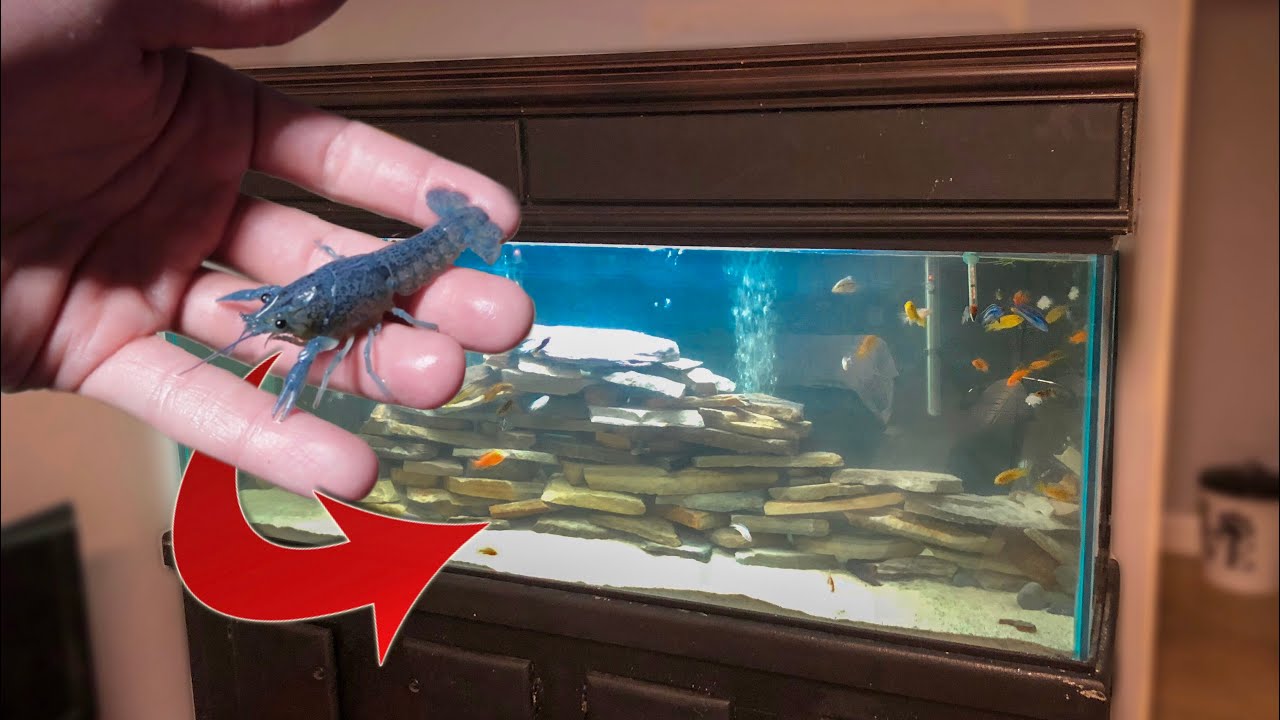In this detailed image, a person's left hand emerges from the left side holding a blue crawfish, which is approximately three to four inches long. A red arrow points from the crawfish to a fish tank in the background, indicating that the crawfish will be placed inside. The fish tank, framed by dark brown wood, is set into a wall with wood paneling and displays various features. The tank bottom is lined with white sand, and several flat rock slabs are stacked to create intricate structures reaching nearly to the top. Among the many fish, which include colorful cichlids in shades of orange, blue, yellow, and white, a large group is congregating in the top right. The tank also contains two bubblers along the back. Outside the tank, there is a visible edge of the wall on the right and possibly a bucket of paint near a door. The fish tank area appears to be part of a cozy, lived-in home, with the brownish wall color providing a warm backdrop.